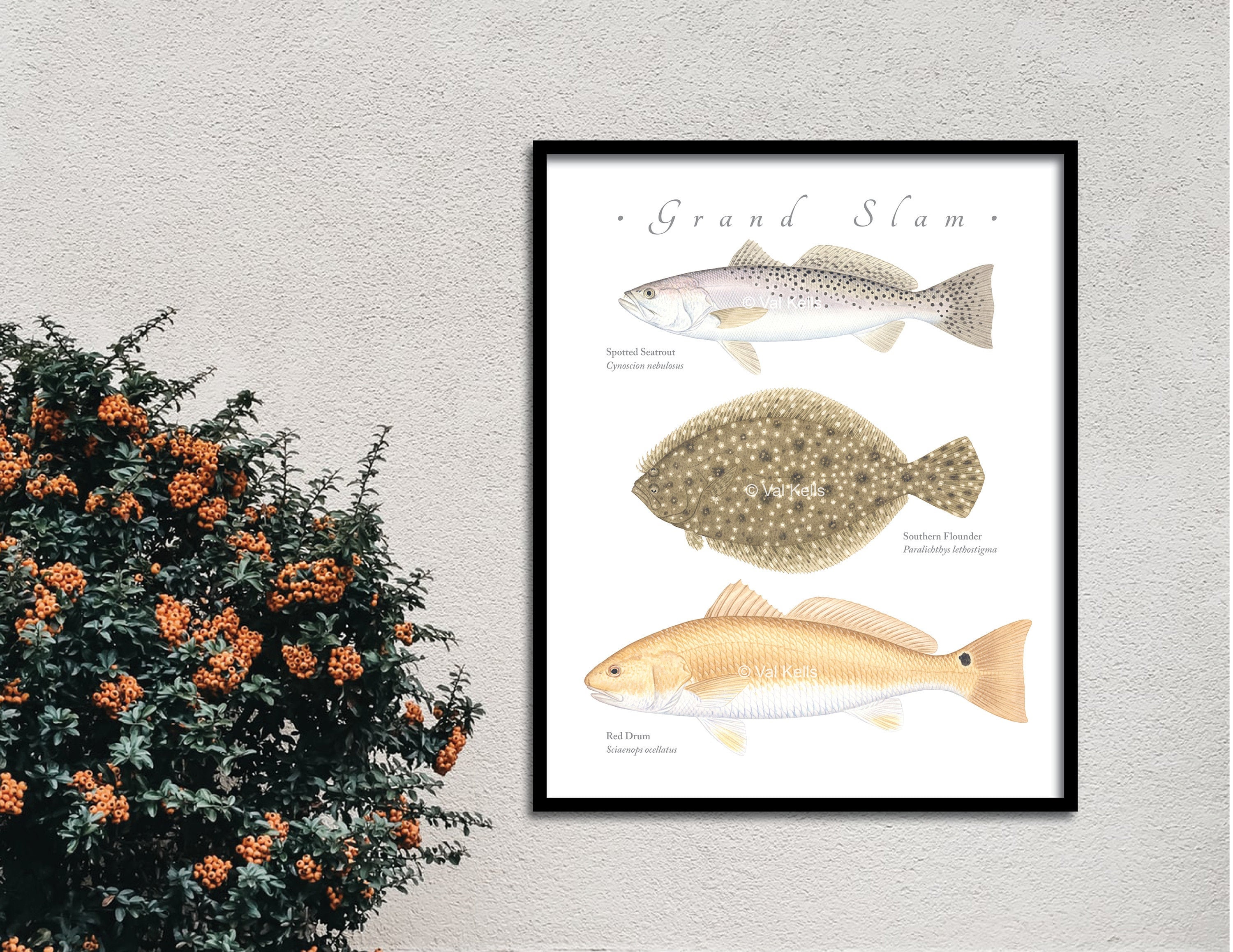The image showcases a framed picture hanging on a textured gray wall, bordered by a sleek black frame. At the top of the frame, the text "Grand Slam" is prominently displayed, bookended by dots and appearing in red and black font. The artwork is signed by Val Kells and contains individual watermarks on each fish.

Below the text, the picture features three fish, all oriented towards the left. The top fish is a gray spotted sea trout (Cynoscion nebulosus), distinguished by its black spots and labeled with both its common name and scientific name. The middle fish is a southern flounder (Paralichthys lethostigma), recognizable by its wide, brown body with black and white spots. The bottom fish is a red drum (Sciaenops ocellatus), characterized by its orange hue on top, a white base, and a distinctive black spot near its back fin.

To the left side of the frame, a large plant with an abundance of green leaves and reddish-orange flowers adds a splash of natural color to the scene.